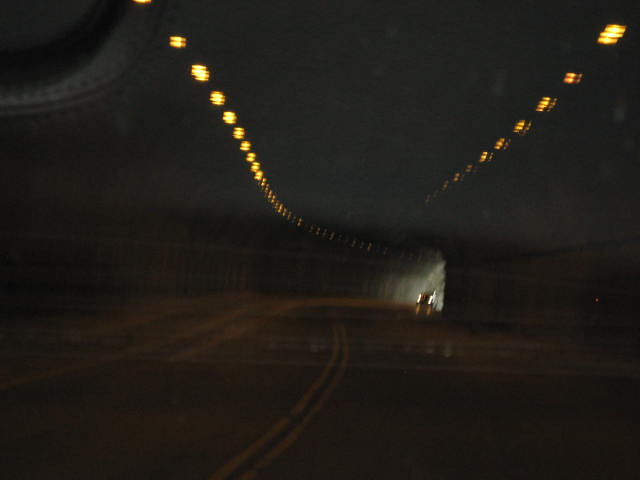A dark car tunnel stretches out before the viewer, illuminated intermittently by rows of dim, orange-tinted lights lining the ceiling. These lights form parallel lines that guide the eye towards the distant exit of the tunnel, positioned at the back right of the image. There, a faint glow from outside daylight seeps in, providing a contrast to the tunnel's shadowy interior. A car, headlights beaming, approaches from this illuminated exit, driving towards the viewer. The image is captured from within another vehicle, evident by the subtle reflections on the windshield and dashboard. Dividing lines on the road are visible, leading the way through the tunnel. In the top left of the image, a partially obscured, round, black object with a white border adds a touch of mystery, hinting at features within the observer's car.